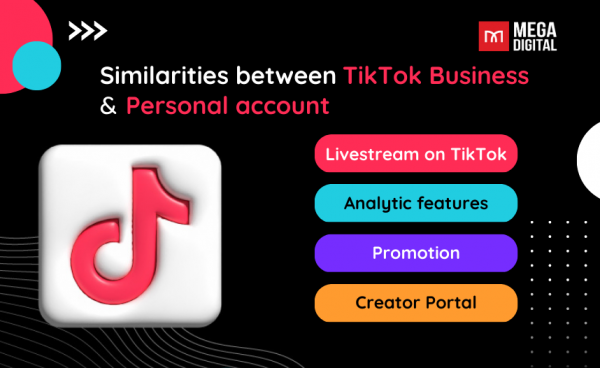**Detailed Caption:**
The image is a screenshot from TikTok featuring a prominent black background with red TikTok symbols encased in white squares. The text "Similar between TikTok business and personal" stands out in bold red lettering, while the accompanying explanation is rendered in white text. The multi-color elements provide additional information: 
- A blue segment with the words "Analytic Features" written in black.
- A purple section displaying "Promotion" in white.
- An orange portion labeled "Creator Portal" in black.

In the top right corner, the words "Mega Digital" are visible alongside half of a white circle. The bottom right corner is adorned with a cluster of small white dots, adding an extra layer of visual interest to the composition.